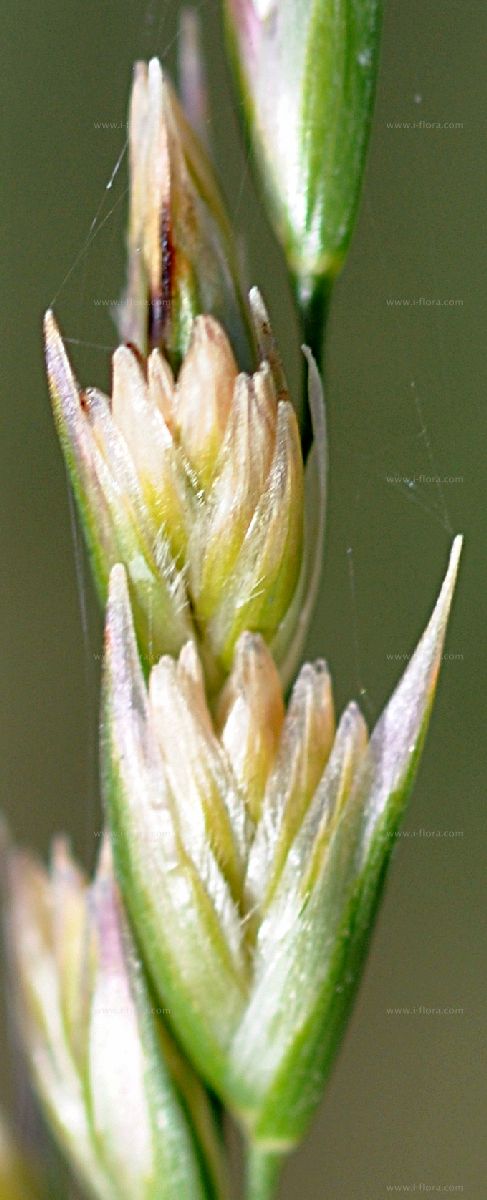The image displays an up-close, detailed view of multiple flower buds against a blurred green background, suggesting surrounding plant life. The flowers, mostly unbloomed, vary in stages of opening and color. The primary focus is on the center, showing a green, slightly open bud revealing pale inner structures tinged with faint pinkish-purple hues. Nearby, there are partially opened yellow flowers with green outer layers and a noticeable dark brown streak running down one side, indicating possible decay. Subtle spider web-like threads interconnect parts of the flowers. Tiny, repeated watermarks from www.i-flora.com are visible across the image, particularly on the slightly unfocused, darker green background transitioning to brown hues at the bottom. The overall image composition is rectangular, oriented vertically, highlighting the intricate and delicate qualities of the flower's structure amidst a not entirely attractive backdrop.